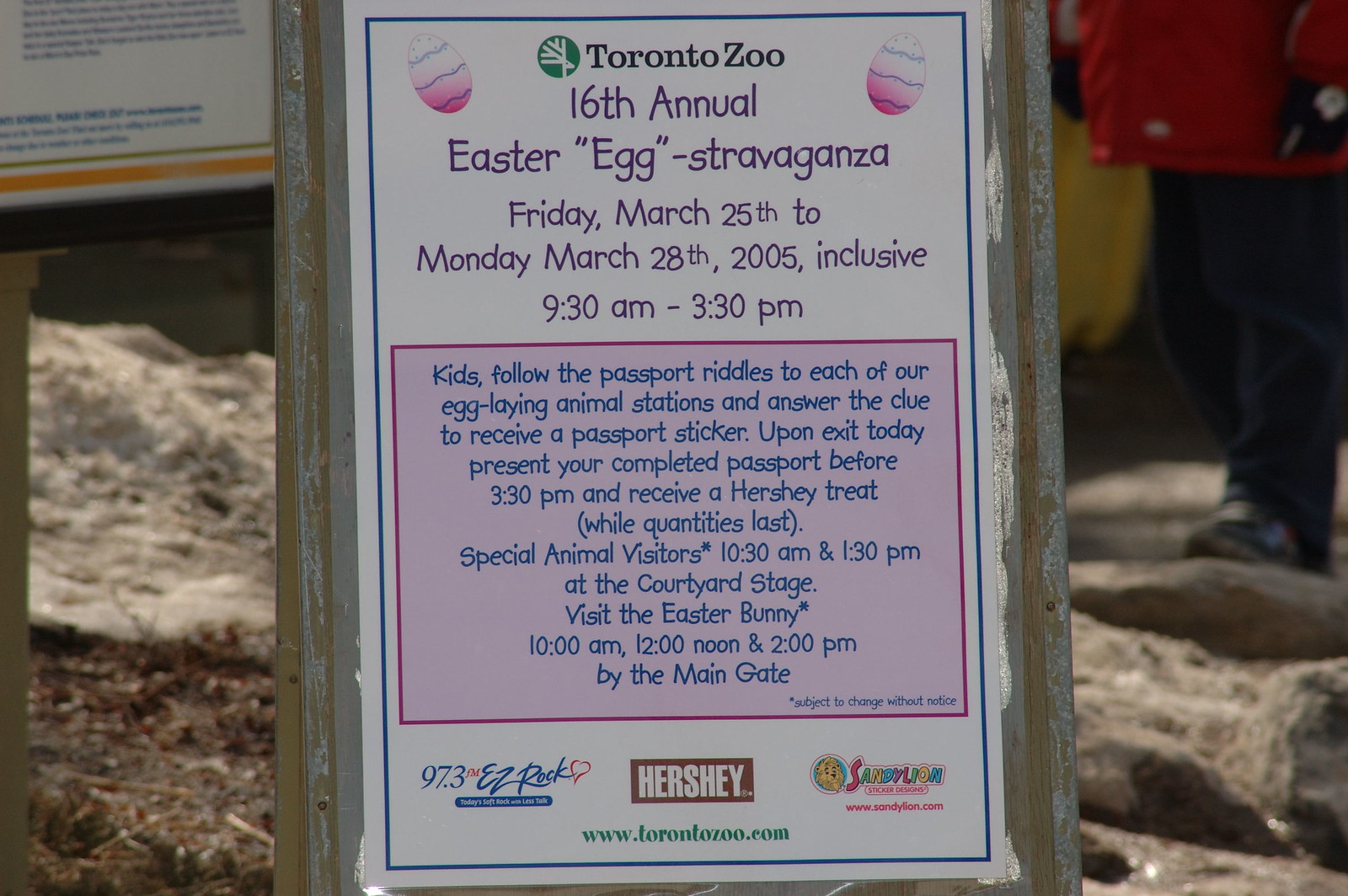The image features a weathered, wooden signage for the Toronto Zoo’s 16th Annual Easter Egg Extravaganza, held from Friday, March 25th to Monday, March 28th, 2005, between 9:30 a.m. to 3:30 p.m. daily. The sign includes detailed instructions for kids to follow the passport trail to various Easter Egg Laying Animal Stations, answer clues, and collect stickers. Upon exiting, participants could present their complete passport at the main gate to receive a Hershey’s treat, while supplies lasted. Special activities included visits from the Easter Bunny, situated near the main gate. The sign itself is detailed with a green serif font "Toronto Zoo" at the top left, accompanied by the zoo's logo. The event details are highlighted within a light pink box bordered by a dark pink line. The base of the sign displays logos for Hershey, a radio station, and potentially a Play Place. The signage, encased in a worn wooden frame, sits on uneven ground amidst twigs, dead grass, rocks, and a barren backdrop, suggesting an outdoor setting. At the bottom of the infographic, the zoo’s website, www.torontozoo.com, is also listed in green serif font.